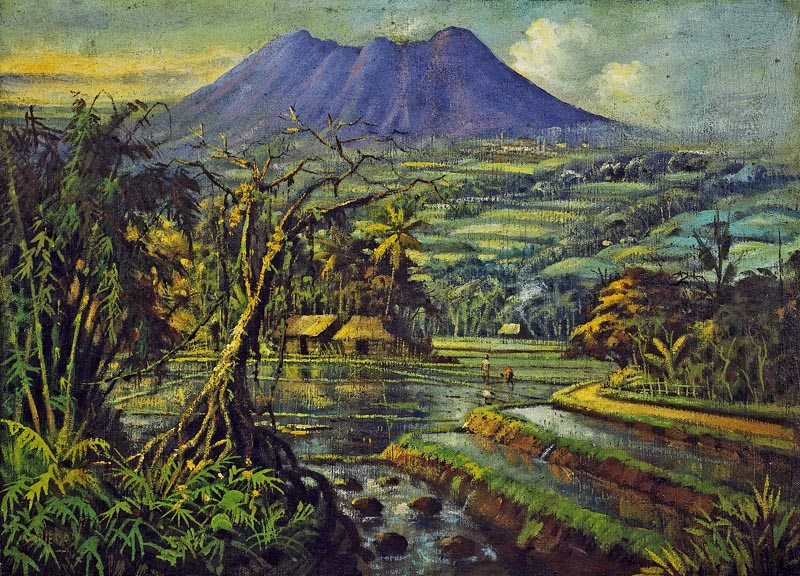This highly detailed painting portrays a serene, jungle-like landscape with a dominant large gray volcano rising in the far distance, framed by a green and blue sky with pockets of white clouds. The foreground is filled with tiered, flooded farmlands that resemble rice paddies, organized in a checkered pattern across the landscape. At the very center of the image stands a brown house adorned with a yellow thatch roof. Surrounding this house is a vibrant array of jungle vegetation, lush with diverse plant life. 

In the fields between the house and the viewer, three people are visible, toiling away in the flooded farmlands: the leftmost person wears a white shirt and brown pants, the rightmost person sports an orange shirt with black pants, and the central figure is clad in a white shirt with gray pants. Flanked by additional tropical foliage and interspersed houses of light tan color with single doors, these elements add depth to the composition. The volcano in the background, with tinges of blues and purples, creates a stark contrast, rising majestically against the lush, predominantly green and yellow tonal setting.